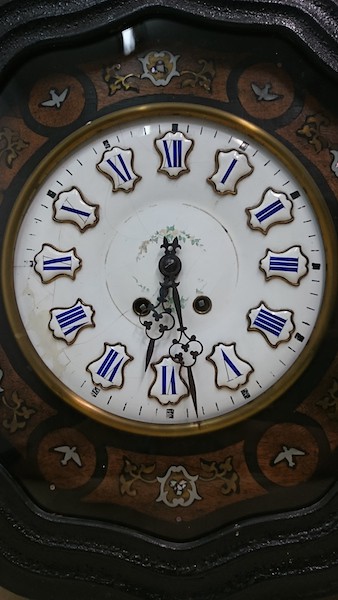This vertically oriented photograph captures a close-up of an antique, ornately decorated clock face. The clock features a white enamel face with blue Roman numerals, each number set against a shield-like background. The minute and hour hands are black, elaborately designed with a floral motif, with the hour hand being shorter. The clock face shows a time of approximately 6:27. Surrounding the white face is a thin gold trim, encased in an intricate bronze rim. Beyond this, the clock's black wooden body is adorned with detailed brown inlaid marquetry, depicting rudimentary motifs of doves, floral elements, and possibly a crest. The inlays appear as though the birds are flying towards the clock face, adding to the vintage aesthetic. The image focuses solely on the clock's face and immediate decorations, leaving the broader setting, support, or positioning of the clock unseen.